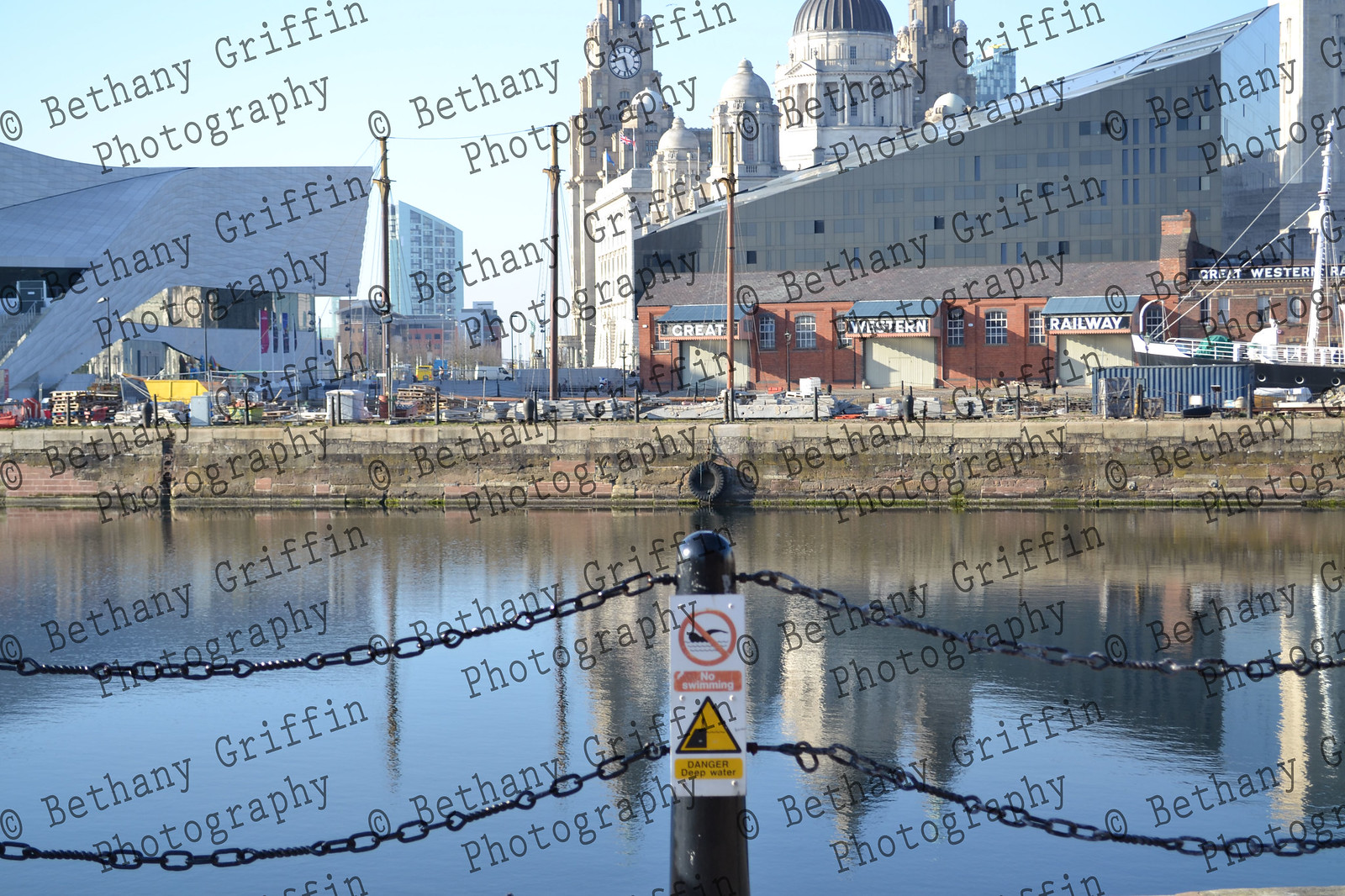This detailed photographic image, captured and watermarked by Bethany Griffin Photography, showcases an industrial waterside scene during daytime. The central focus is a still canal bordered by a concrete wall from which a pipe protrudes, potentially expelling sewage. Reflective waters mirror the striking architecture that comprises the backdrop. Dominating the scene is a red brick warehouse emblazoned with "Great Western Railway." Next to it, a majestic clock tower, indicating the time as almost 8:30 AM, rises alongside a grand church with imposing gray domes. Adjacent to the warehouse, a sleek concrete modern building contrasts with the historic structures. Industrial supplies are scattered along the dock in front of the railway building, and a boat with a single mast is moored nearby. Framing the foreground, a chain-link barrier, held by small black poles, carries cautionary signs, including a yellow triangle warning "Danger, Deep Water" and "No Swimming." Further enhancing the urban-industrial contrast, a massive glass building can be seen behind the church, suggesting a bustling urban center beyond the quiet canal. Streetlights dot the pathway along the water, completing this vivid blend of natural tranquility and manmade utility.